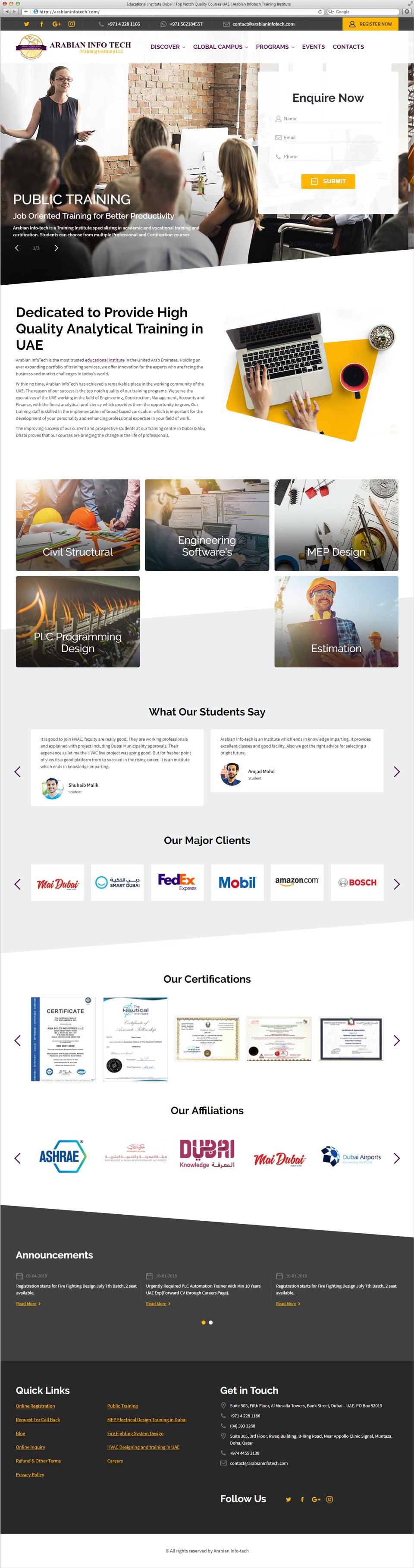**Detailed Caption:**

The advertisement consists of five distinct sections, each meticulously designed to convey various aspects of a professional training program. 

1. **Instructor and Call to Action:** The topmost section features an image of a lady, presumably an instructor, passionately teaching a class. A prominent "Enquire Now" button suggests an invitation to prospective students. The text below announces, "Public Training," indicating an open invitation for enrollment.

2. **Commitment to Quality:** The subsequent section proudly declares, "Dedicated to Provide High-Quality Analytical Training in UAE." It is visually supported by an icon resembling a geometric shape integrated with a typewriter. The scene is thoughtfully enhanced with two hands poised for typing and a cup of coffee resting on the platform, symbolizing a focused learning environment.

3. **Visual Representation:** Following this, a segmented area displays six squares. The top row's first three squares contain diverse images, adding visual interest, whereas the bottom row reveals two images flanking a central blank square, creating a balanced yet intriguing layout.

4. **Student Testimonials and Clientele:** The fourth segment is divided into sharing testimonials under "What Our Students Say," complete with student text and images, reflecting personalized feedback. Adjacent to this, "Our Major Clients" spotlight prominent company logos such as FedEx, Mobile, and Bosch, illustrating the program's reputable affiliations.

5. **Certifications and Affiliates:** Progressing further, "Our Certifications" showcases the array of certifications the program holds, emphasizing credibility. Near the end, "Our Affiliates" is listed, displaying the program's collaborative networks.

6. **Contact and Engagement:** The final segment, distinguished by a black geometric shape, directs viewers to "Quick Links," and encourages engagement through "Get in touch" and "Follow us," ensuring straightforward navigation and fostering connectivity.